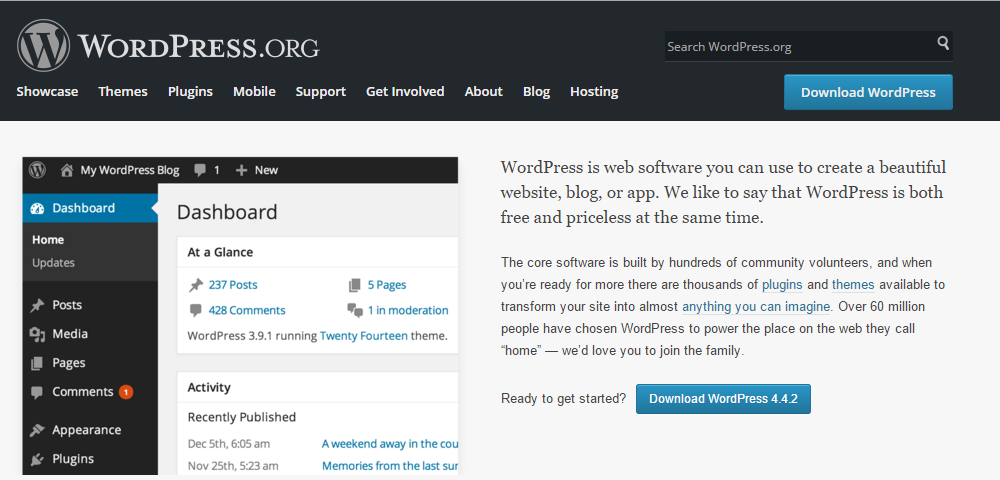The image features the homepage of Wordpress.org, prominently displayed within a sleek black box. At the top, the Wordpress logo, a distinctive 'W' enclosed in a circle, is clearly visible. Adjacent to this logo is a search bar labeled "Search wordpress.org."

Below the search bar, a navigation menu lists the following options: Showcase, Themes, Plugins, Mobile, Support, Get Involved, About, Blog, and Hosting. A noticeable blue button labeled "Download WordPress" stands out against the page's backdrop.

The section beneath the button reads: "Wordpress is web software that you can use to create a beautiful website, blog, or app. We like to say that WordPress is both free and priceless at the same time." This introductory text skips a line to further elaborate: "The core software is built by hundreds of community volunteers, and when you're ready for more, there are thousands of plugins and themes available to transform your site into almost anything you can imagine. Over 60 million people have chosen WordPress to power the place on the web they call home. We'd love for you to join the family."

Further down, a call-to-action invites users to start their journey with a second blue button that reads "Download WordPress 4.42." On the left side of this call-to-action, a sidebar provides a glimpse into the dashboard's overview, which includes "At a Glance," revealing there are 237 posts and 428 comments.